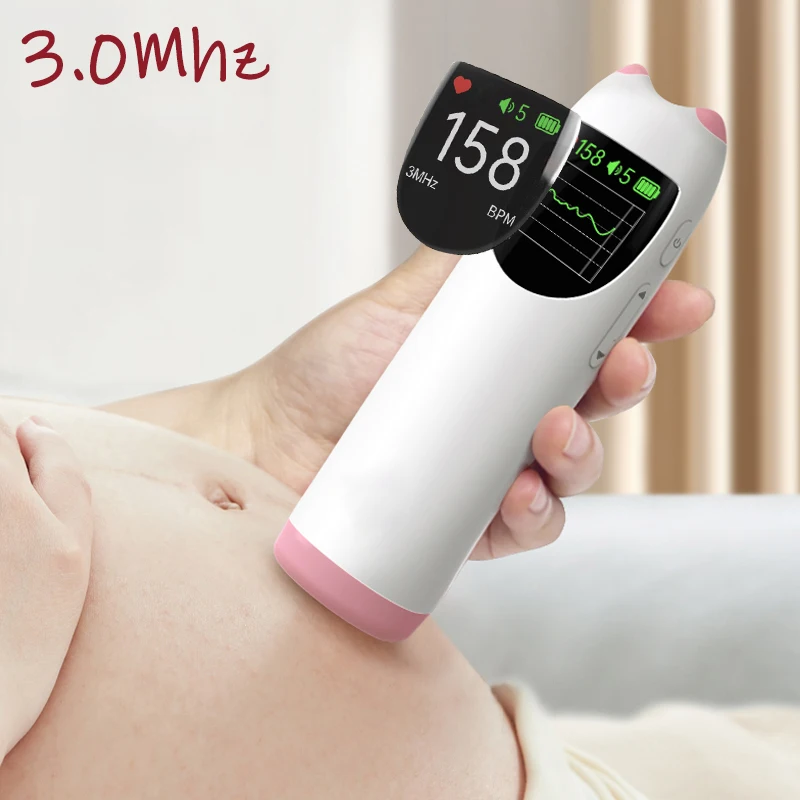In the image, a pregnant woman with fair, light skin holds a medical device to her large belly, using her left hand to position it. The device, primarily white with pink ends, is oval and rectangular, featuring small pink accents at the top. The display on the device shows a reading of "158," likely indicating the baby's heartbeat in beats per minute (BPM), with "3.0 MHz" noted in red letters. At the top left of the screen, there is a red heart icon suggesting that the device is measuring the baby's heartbeat. Other display elements include a speaker icon marked with a "5" for volume and a battery indicator. There are up and down arrows along the side of the device, likely for controlling the volume or navigating settings. The woman's belly shows a prominent pregnant shape, complete with a visible belly button and the linea nigra, the dark line running up her abdomen. Her fingernails are unpainted, and the image also includes a magnified view of the device's screen for clarity.